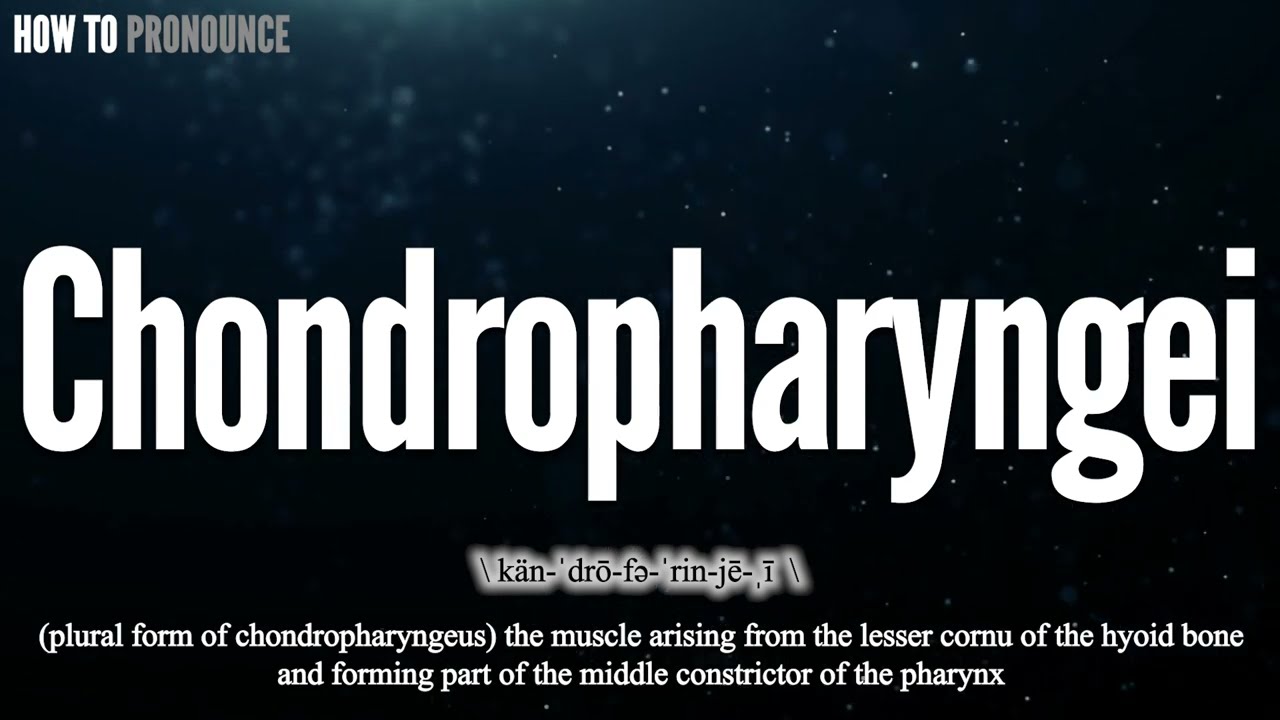The image features a large piece of white text that spans the width of the frame, centered against a dark, nebulous background reminiscent of space filled with specks of light, though it's clearly abstract. In the upper left corner, there's small text reading "how to pronounce" near a faint blue hazy glow. The main text in bold letters spells out "C-H-O-N-D-R-O-P-H-A-R-Y-N-G-E-I," and directly beneath it is a phonetic transcription, detailing the pronunciation intricately, akin to dictionary entries. Additionally, under the phonetic guide, there is a smaller line of text that describes the word as the plural form of "chondropharyngeae," and further explains that it refers to a muscle originating from the lesser corneal of the hyoid bone, part of the middle constrictor of the pharynx.